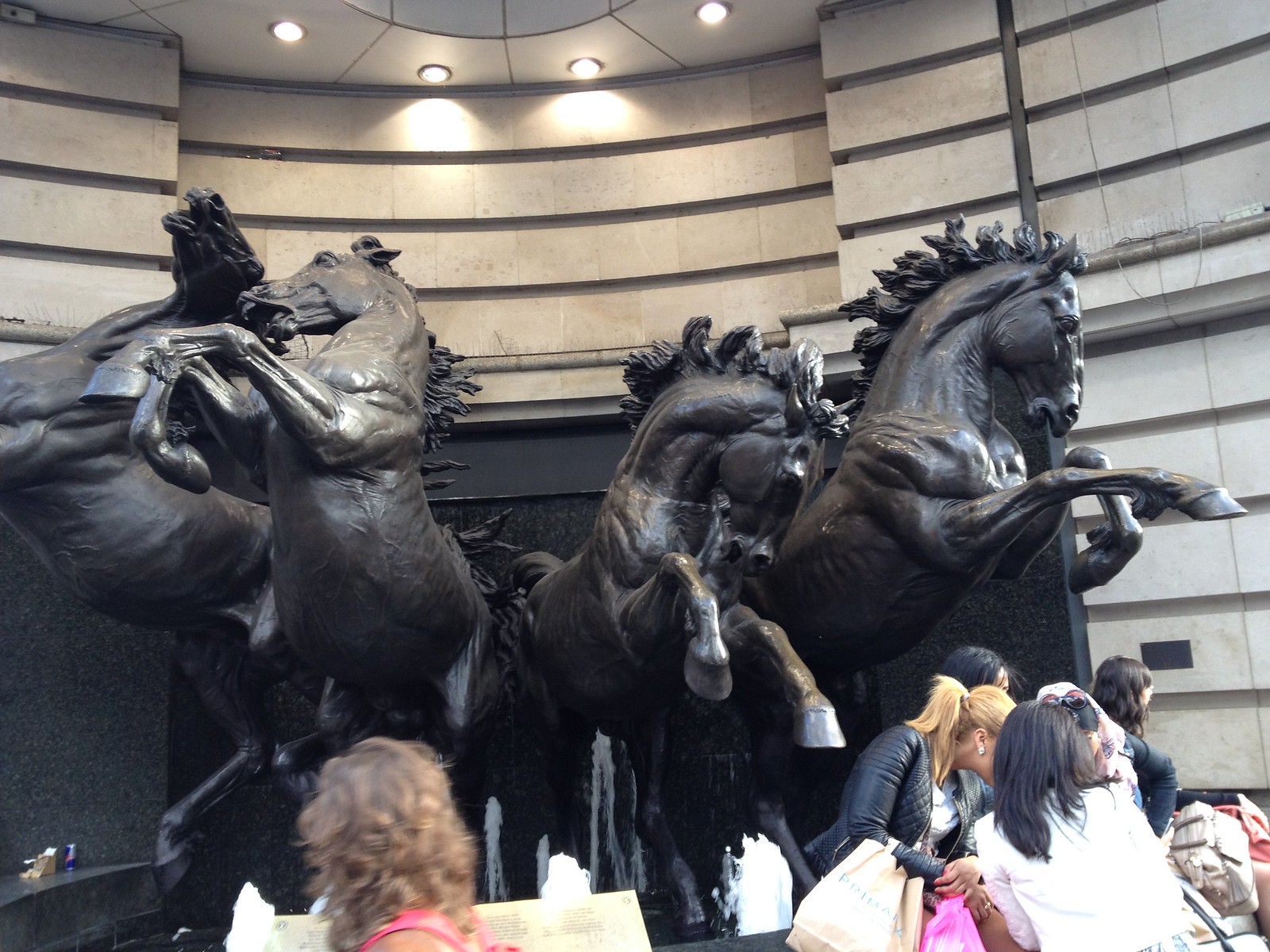This photograph captures a striking sculpture of four horses, which appears to be crafted from a dark, potentially metallic material like bronze, black granite, or black onyx. The horses are dynamically posed, rearing up on their hind legs with distressed expressions and some possibly holding bridles in their mouths. They seem to be emerging or galloping from a curved, wall-mounted backdrop that features horizontally aligned white planks with black lines.

The scene includes a fountain in front of the sculpture, with little spurts of water adding to the dynamic setting. The location appears to be an exterior covered area adjacent to a larger building. Above the sculpture, four built-in ceiling lights illuminate the display, along with bright fluorescent bulbs.

A crowd of people is gathered around the fountain. In the foreground, a person with blonde hair in a ponytail is visible from the side, and another with brown hair, wearing a brown top and a pink backpack, is seen walking to the left, apparently near a plaque. Several other individuals are seated on the edge of the fountain, some holding shopping bags, indicating they might be taking a break from sightseeing or shopping. In the bottom left of the image, someone has placed a Red Bull can and a sandwich. Overall, the scene is bustling with activity and draws attention to the imposing, rearing horse sculptures.